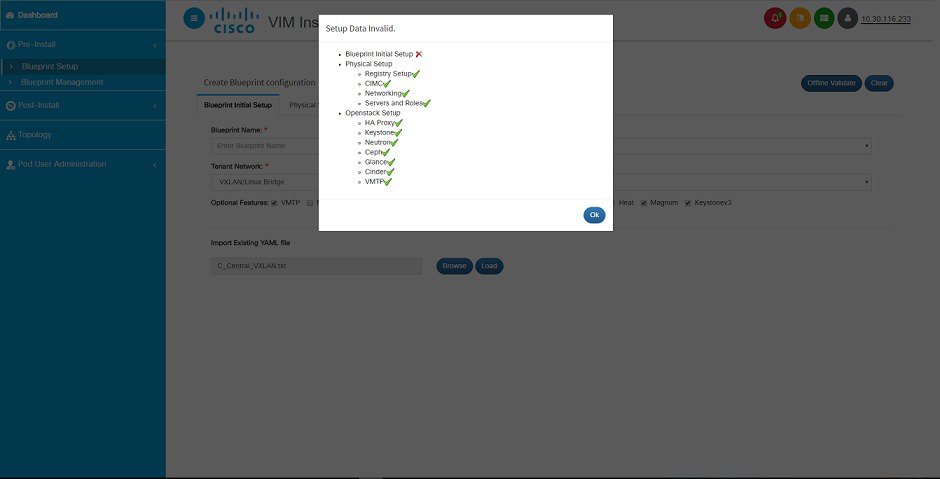Here's a cleaned-up and detailed caption for the image:

The screenshot depicts a section of the Cisco website, showcasing a detailed setup process with various status indicators. At the forefront, a box is highlighted with a red cross next to "Initial Set Up," signifying invalid data. Other setup stages are displayed with green ticks, indicating successful completion: "Physical Set Up," "Registered Set Up," "CIMC," "Networking," "Service and Roles," "OpenStack Set Up," "HAProxy," "Keystone," "Neutron," "Ceph," "Glance," "Cinder," and "VMTP." 

An 'OK' button at the bottom allows the user to dismiss the highlighted box. In the background, a blue column runs down the left-hand side featuring a dashboard with various clickable options: "Pre-Install," "Blueprint Set Up," "Blueprint Management," "Post-Install," "Topology," and "User Administration," each potentially offering additional drop-down menus. 

The upper right corner shows color-coded notification buttons: a red notification button, along with amber, green, and purple buttons whose contents are partially obscured. Additional functional buttons such as "Offline Validate," "Clear," and "Browse" are also visible on the interface. The Cisco VIM logo and the partially obscured text "INTS" are located at the top of the page.